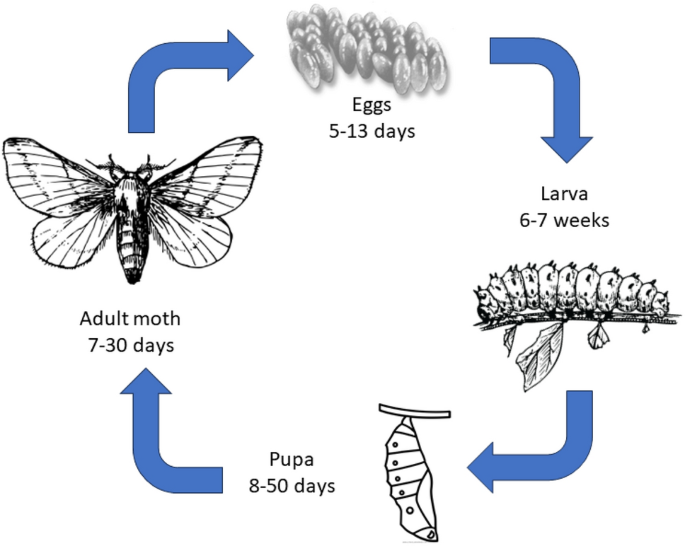This black-and-white diagram illustrates the life cycle of a moth, showcasing four distinct stages arranged in a square pattern, each connected by curved blue arrows. At the top center, labeled "Eggs (5-13 days)," is a detailed illustration of a cluster of oval eggs. The cycle progresses to the right and downward to the "Larva" stage, depicted as a caterpillar on a plant stem, marked "6-7 weeks." Continuing downward and to the left is the "Pupa" stage, represented by a simple, line-drawn chrysalis hanging from a branch, labeled "8-50 days." Finally, moving upward and to the left is the "Adult Moth" stage, showing a top-view of a fully developed moth with wings spread, labeled "7-30 days." Each arrow guides the viewer through the stages, ultimately looping back to the eggs to indicate the continuous nature of the moth's lifecycle.